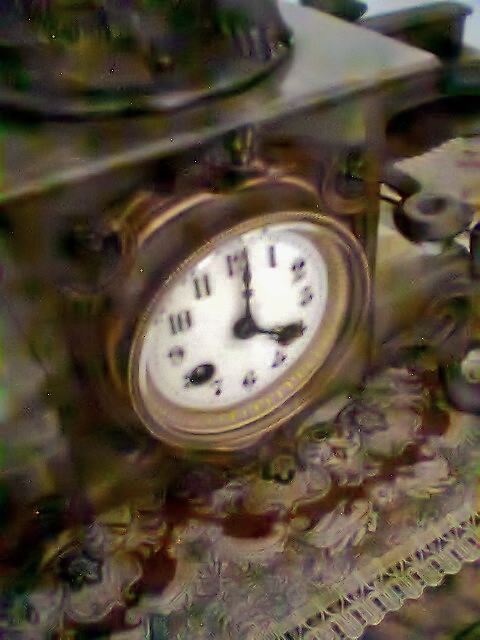In this image, we observe a very blurry photograph of a clock, seemingly taken indoors. The clock is set upon a placemat made of fabric adorned with ornate floral embroidery. The clock is mounted on the side of a square wooden box, crafted from dark wood, though the full extent of the box is not visible. The clock itself features a round, copper-colored housing with a white face displaying black numbers and hands. The image contains no text.